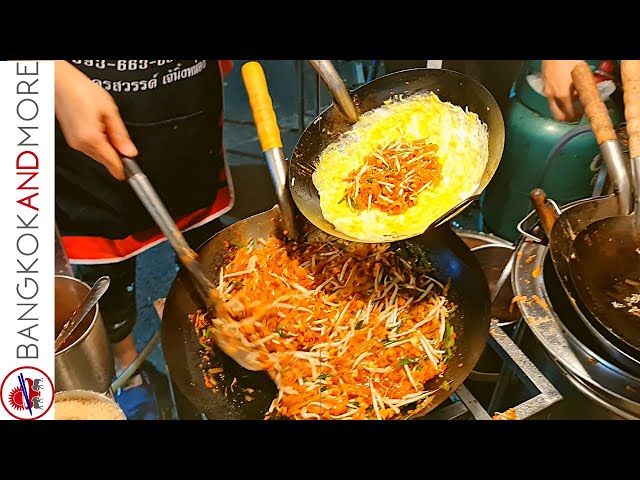The image is a full-color, landscape-oriented photograph bordered by thick black margins at the top and bottom and a white border on the left side featuring the text "Bangkok and more" in large, thin capital letters, with a round logo of chopsticks above it. The scene depicts an outdoor cooking setting, possibly in Thailand. The focal point is a chef in a black apron with white writing in Thai. The chef is using two frying pans for wok-style cooking. One hand is visible on the right side, suggesting the presence of another person. The smaller pan, held above the larger metal pan, contains an egg mixture with rice and cheese. The larger pan, on the flame, holds red rice, more cheese, and possibly bean sprouts with green herbs. Surrounding the central wok are stacks of other woks, adding to the busy, culinary atmosphere.